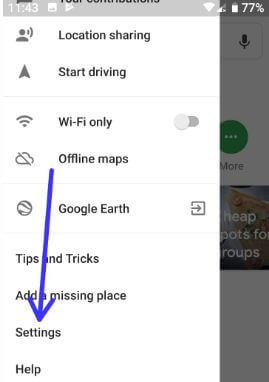A screenshot taken from a smartphone display. At the top-left corner, the time is shown as 11:43 AM, while the top-right corner displays the battery level at 77%. The main portion of the screen features a white interface with a list of options:

1. At the very top, there's an icon of a person with lines beside their face, labeled "Location sharing".
2. Below that is an upward-pointing arrow next to the text "Start driving".
3. The next option reads "Wi-Fi only" with a toggle switch to turn it on or off.
4. Following this, there's a cloud icon with a cross through it, labeled "Offline maps".
5. Beneath this is a circle with two lines through it, indicating "Google Earth" with an arrow pointing to the right.
6. Next in the list are "Tips and tricks" and "Add a missing place".
7. The subsequent option is "Settings," highlighted by a blue arrow drawn next to it.
8. The final option at the bottom of the list is "Help".